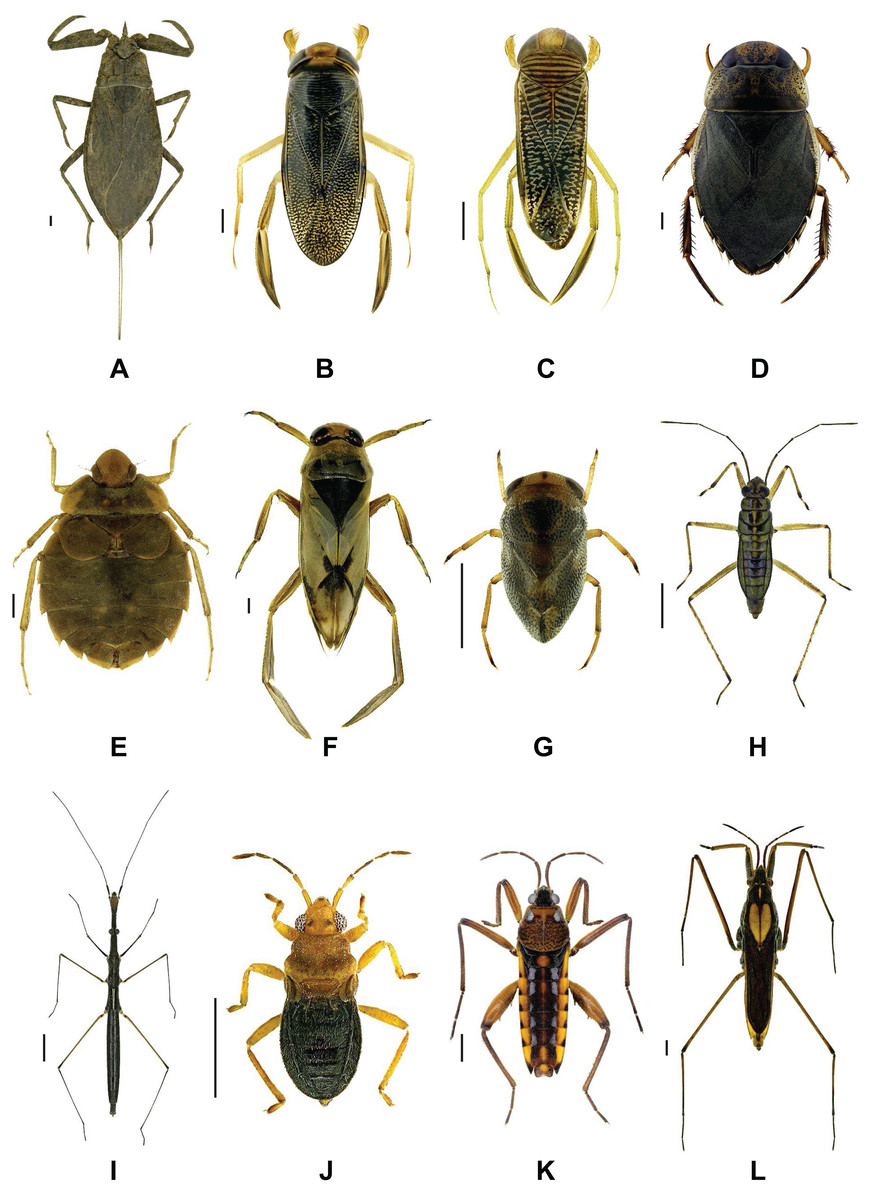This image features a neatly arranged collection of 12 insect photographs, positioned against a solid white background. The insects, showcasing a variety of species including beetles, cockroaches, stink bugs, and crickets, are laid out in three rows of four, labeled from A to L. Each insect is photographed from an above perspective, allowing for a clear view of their distinctive features and colors, ranging from dark browns and blacks to yellows and greens. One notable insect has a very round, oval body with a pointy bottom, spiky sides, pincers at the head, and stubby legs, predominantly black in color. Another insect resembles a tick, sporting a jagged-edged, round shell in brownish-green hues with thin yellow legs. There's also a slender, elongated insect similar to a stick bug, all dark gray with long, thin legs and antennae. This detailed arrangement appears to serve as a scientific reference, likely for educational purposes.